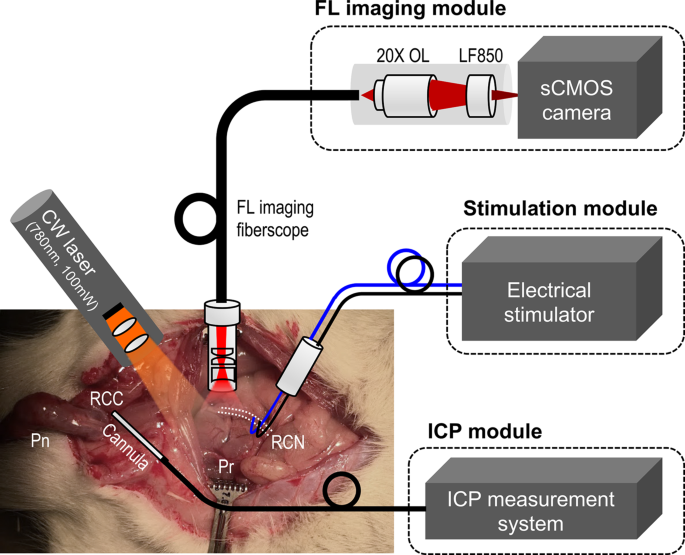The image is a detailed illustration of surgical equipment and procedures, featuring both a photograph and various diagrams. The left side showcases a photograph of surgery being performed on an animal with white fur, where retractors are used to hold open an incision, exposing the underlying tissues. Various elements are labeled in the photo, including 'canola' leading to an ICP module, which indicates an ICP measurement system. Above this section, 'CW laser' is noted.

On the right side, the diagrammatic portion includes multiple labeled components. At the top, 'FL Imaging Molecule' is displayed, followed by a labeled image '20X 0OL LF850.' Below this is an image of a tube channeling red light through two parts. There is a black 3D box labeled 'SCMOS Camera,' followed by another black 3D box labeled 'Simulation Module.' Additionally, purple and black lines link parts of the diagram to a square labeled 'Simulation Module,' highlighting various connections, including to an electrical stimulator. The comprehensive display ties together advanced imaging and functional modules utilized in the surgical process.